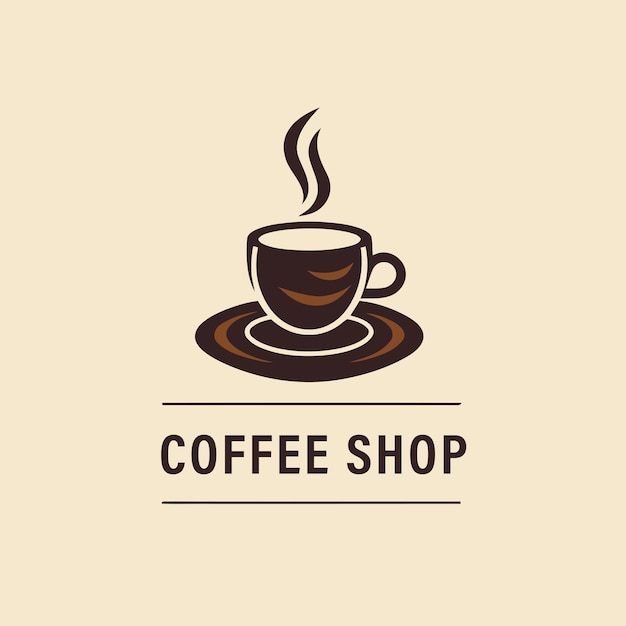The image features a simple, yet detailed logo set against a beige background. At the center of the logo, a dark brown coffee cup rests on a saucer. The saucer is designed in a cartoon style and exhibits a lighter brown inner circle surrounded by a dark brown outline, with additional medium brown accents on either side. The coffee cup itself, similarly dark brown, includes two tan, crescent-shaped accents on its exterior, resembling upside-down smiles. Rising from the cup are two brown, swirl-shaped lines, symbolizing steam. Underneath the cup, there are two thin, dark brown lines — one above and one below — framing the text "COFFEE SHOP" written in capital letters. The overall design uses varying shades of brown to create depth and visual interest.